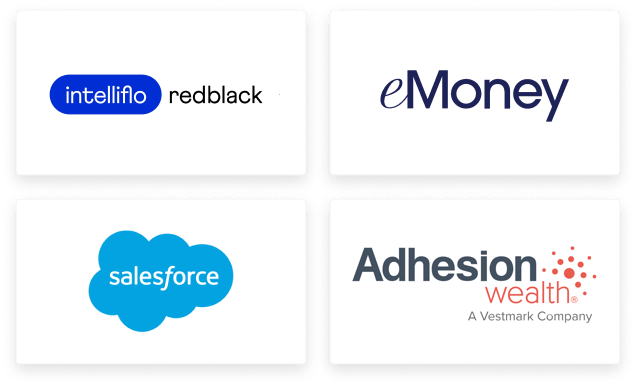The image features four distinct company logos, each placed within its own square box accentuated by a shadow effect.

1. The first logo belongs to Intelphilo. It is designed in a red and black color scheme. The name "Intelphilo" is portrayed within a circular shape, featuring blue with white lettering, while "red-black" is displayed in simple black letters.
   
2. The second logo represents e-money. The "e" is styled in a unique font, differing from the font used for "money."

3. The third logo is for Salesforce. It is depicted as white lettering within a cloud shape, reminiscent of how a child might draw a cloud. Notably, the "f" in "force" is in a different font from the rest of the word.

4. The fourth logo is for Adhesion Wealth, a Vestmark company. In this logo, "Adhesion" is the most prominent element, portrayed in bold black font. "Wealth" is written in a thinner, red font, while "a Vestmark company" is in a similar thin font, but in a gray-black color. Additionally, the logo features an icon resembling a sun, consisting of a central circle surrounded by two layers of six smaller circles each.